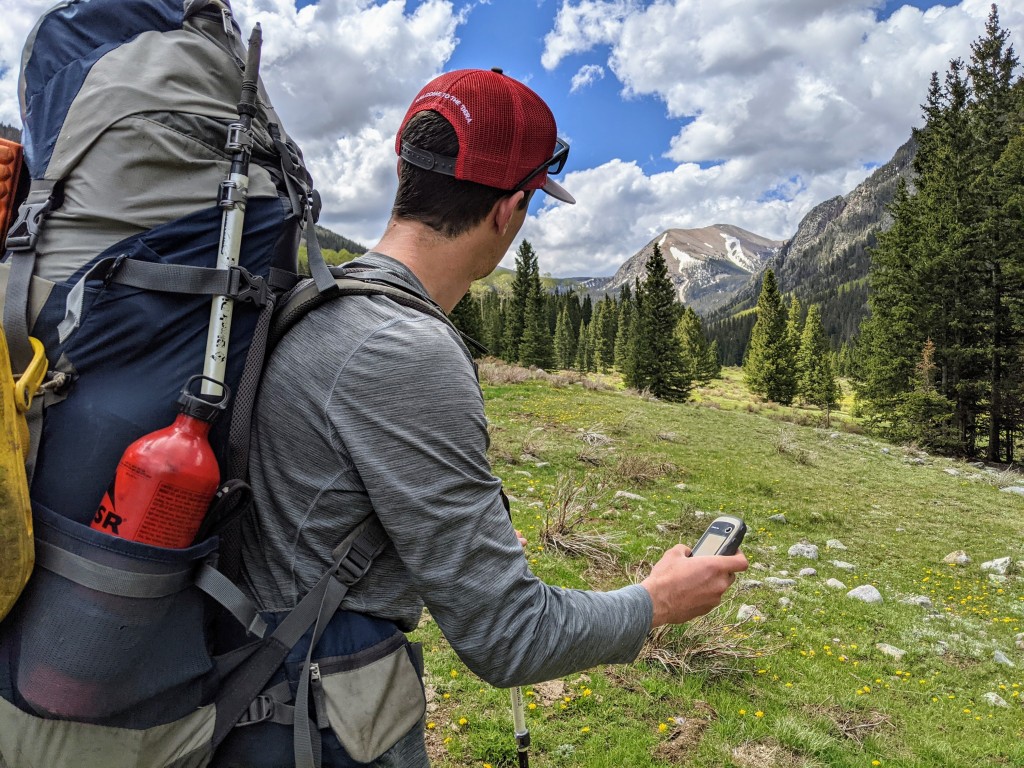The image is a promotional photograph featuring a hiker in a wilderness setting, with majestic mountains in the background under a blue sky dotted with fluffy clouds. The hiker, a man, is turned away from the camera and looking towards the mountain range. He is standing on a green hill spotted with dandelions and adorned with small stones, suggestive of a springtime setting. Trees can be seen in front of his line of vision, enhancing the natural scenery.

The hiker is wearing a red baseball cap with sunglasses perched on its brim, a gray sweatshirt made for hiking, and blue pants. He is carrying an enormous, heavy-looking hiking backpack that extends higher than his head, featuring a blue color with gray stripes. Attached to the backpack is a prominent red water bottle placed in a front-facing pocket.

In his right hand, he holds a GPS tracker or emergency communication device, underscoring the preparedness for his outdoor adventure. Additional gear is visible, including hiking sticks fastened to the backpack and a pair of Crocs. This comprehensive ensemble highlights the hiker’s readiness for an extended trek or camping expedition in the serene woodland and mountainous environment.